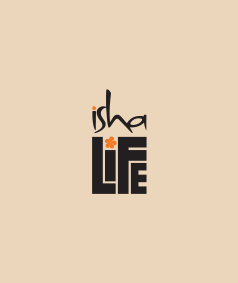The image is a simplistic square logo set against a light beige background, featuring the words "Isha Life." The word "Isha" is written in a very thin, stylized, almost freehand black script with an orange dot atop the "i." Below it, the word "Life" is depicted in large, dark block letters with a unique design where the "L" and "F" both overpower and partially overlap the smaller "i" and "e." The "i" in both "Isha" and "Life" is dotted with an orange element, appearing as a dot in "Isha" and possibly a small star or flower in "Life." The "e" in "Life" is notably smaller and confined beneath the crossbar of the "F," fitting into the space created by the surrounding letters like a puzzle piece.